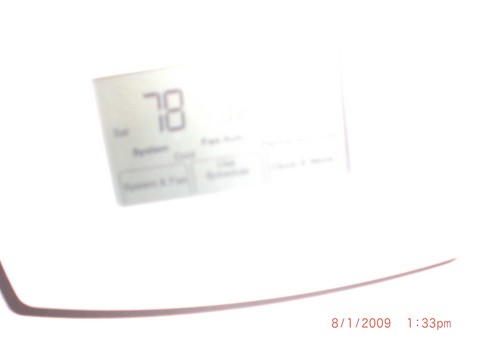The image appears to be a highly degraded printout, likely from a fax machine, photocopier, or inkjet printer with depleted ink. The print condition suggests it has been subjected to significant fading, possibly due to prolonged exposure to sunlight. At the bottom of the page, a digital-style text reads "8-1-2009 1:33pm," indicative of an older timestamp. Above this text, a vertical black line and a dark smudge stretch across the page, further evidencing the poor print quality. Dominating the center of the image is a display, possibly from a central heating system, showing the large number "78." Surrounding this central display, faint boxes and text are visible but too blurred to decipher. The overall quality of the image is severely compromised, making it difficult to ascertain further details.